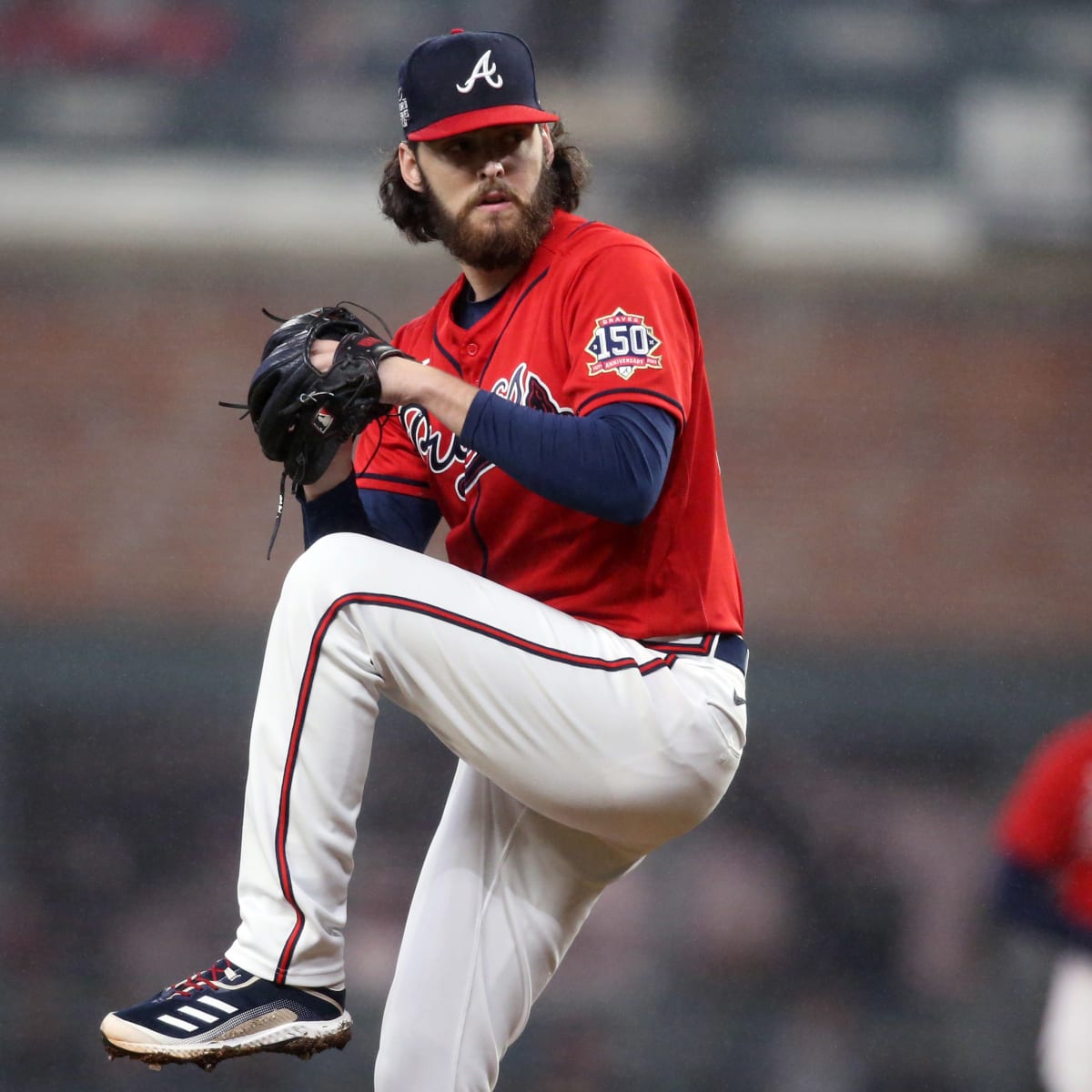This image captures a professional baseball pitcher mid-action, poised to throw the ball with his left leg raised. He sports a serious expression, accentuated by his slightly long, curly brown hair that falls just above his shoulders and a thick brown beard. The player is clad in a striking red or orange and navy blue jersey detailed with the team name—possibly the Orioles—though partially obscured by his arm. Notable on his left sleeve is a white patch with the number "150." Underneath his jersey, he wears a blue long-sleeve shirt. His white pants are highlighted by a red stripe running down each leg, complemented by a dark blue belt. The pitcher's navy blue and white Adidas shoes feature distinct red shoelaces and the iconic three-stripe logo. He wears a navy blue cap with a large white "A" and a red brim. In the blurred background, the stands of a stadium are visible, filled with spectators, and another player can be partially seen in the lower right corner of the image.